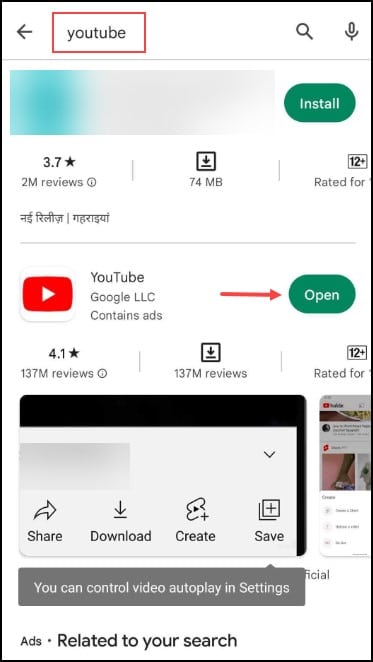In this detailed screenshot, we see a user interface for the YouTube app. On the left side, an arrow points to a highlighted "YouTube" logo enclosed in a red square. Adjacent to this is a magnifying glass icon, indicative of a search function, and a microphone icon, usually for voice searches. A thin gray line separates these elements from a gradient-colored area below.

Within the gradient section, there is a prominent green button labeled "Install." Accompanying this are user ratings—3.7 stars based on 2 million reviews—and an indication that the app is rated suitable for users aged 12 and above. 

Further down, another gray line leads to a segment displaying the text "YouTube, Google LLC." An arrow here points to a green "Open" button. The YouTube logo is also present in this section, reinforcing the app's branding.

Additional details include a 4.1-star rating garnered from 137 million reviews. An arrow directs attention downward towards another age rating of 12+. Below this, in a gray area, is a pop-up box with options to "Share," "Download," "Create," and "Save" content related to the user's search. This box is bordered by a thin black line, emphasizing its interactive functions.